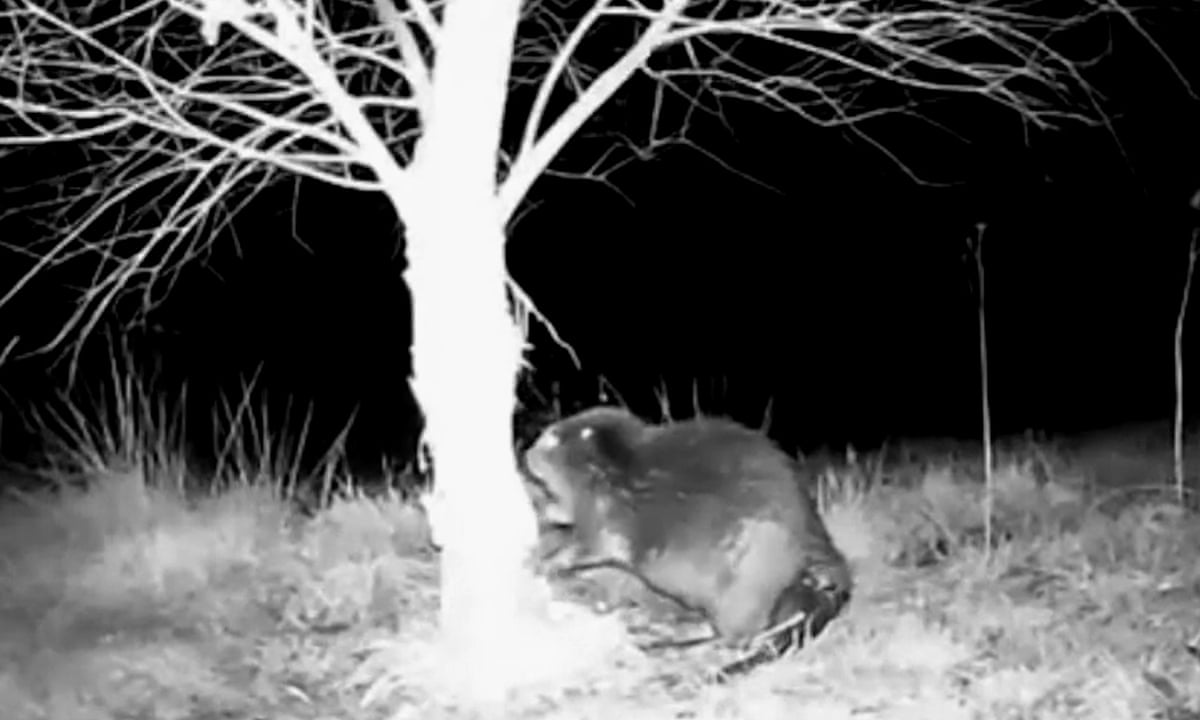This monochrome, night vision image, likely captured by a motion-sensing trail camera, features a striking scene in a wooded area at night. A brilliant flash illuminates the scene, whiting out the bare tree at the center, highlighting its trunk and branches in stark white against the darkness. At the base of this tree stands a beaver, its reflective eyes caught in the light, giving it an eerie appearance. The beaver appears to be touching the tree with its paws, possibly preparing to gnaw on the trunk. Surrounding the tree is a landscape of short grass, with some taller patches interspersed, and the entire setting exudes the bare, empty feeling of winter. The overall image captures a solitary moment in nature, rendered in shades of black, white, and gray.